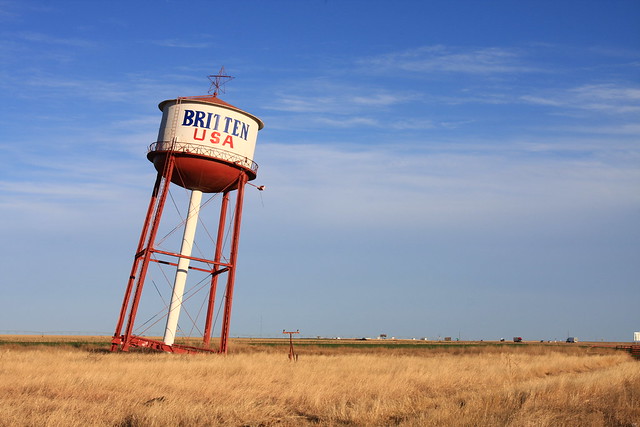This vividly detailed photograph captures a vast, prairie-like expanse characterized by swathes of tan and beige grasses stretching across the bottom fifth of the image. The scene evokes the open plains, possibly of North Dakota, Nebraska, or Kansas. Above, the sky transitions from a light blue near the horizon to a deep, clear blue at the top, interspersed with streaks of thin, wispy white clouds.

Dominating the left side of the photograph is an old, tilted water tower, precariously leaning to the right, more dramatically than the Leaning Tower of Pisa. The structure stands on four rust-red legs, with a central white pipe that either feeds into or drains the tank. This cylindrical tank is ringed by a red metal walkway and topped with the same rust-red color. The main body of the tank is off-white, emblazoned with the name "BRITTEN" in large blue letters, and "USA" beneath it in red. Atop the tank, an antenna protrudes modestly, alongside a small, five-pointed star, adding a touch of rural Americana to the scene. In the distant background, faint outlines of buildings or constructions are visible, adding depth and context to this quintessentially Midwestern landscape.